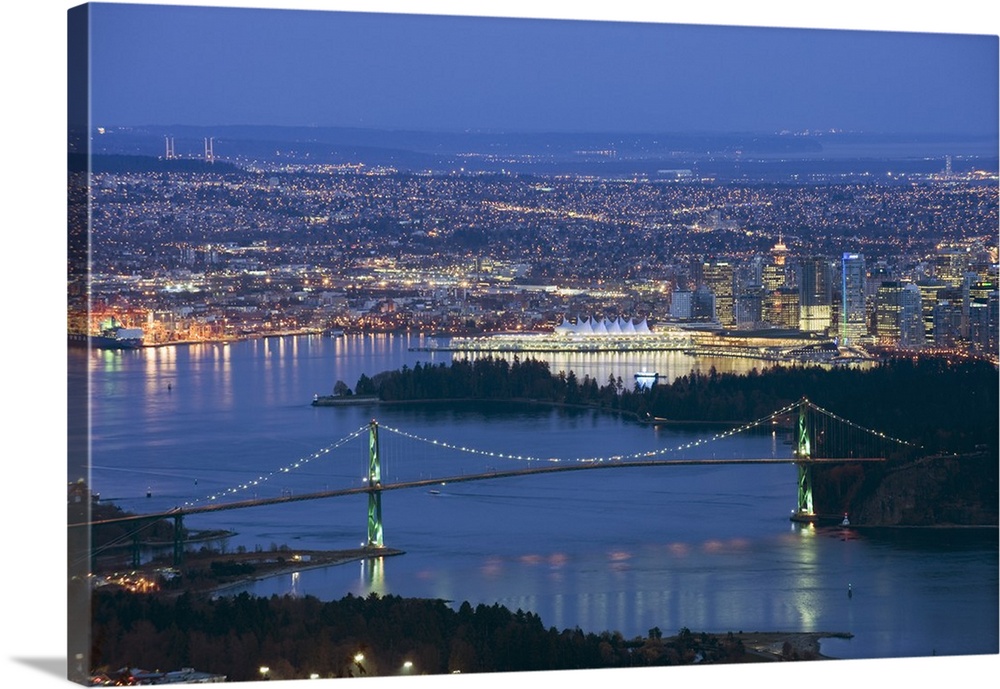This photograph captures a stunning nighttime aerial view of a bustling city set against a backdrop of rolling hills and a hazy, twilight sky transitioning to night. Dominating the central foreground is an expansive body of water, possibly a bay or river, reflecting the myriad lights of the city. A prominent suspension bridge, its pillars tinged green and adorned with festoon lighting, stretches across the water, guiding the eye towards the cityscape beyond.

The city itself is vibrant and well-illuminated, with numerous tall skyscrapers, particularly clustered on the right side, and a notable, uniquely designed building in the center that hints at an iconic structure, perhaps reminiscent of the Sydney Opera House. The skyline is a mix of towering buildings and smaller structures, evoking a sense of a densely populated urban area. To the left, there is a particularly bright patch that further highlights the city's dynamic aura.

In the foreground, lush trees with abundant leaves suggest a setting amid spring or summer, while the presence of a peninsula adds an intriguing element to the composition. The scene is intricately detailed, with electric lights casting shimmering reflections on the water and illuminating the city's architectural diversity. The rolling hills in the background envelop the city in a natural embrace, completing this captivating vista of urban and natural beauty intertwined.